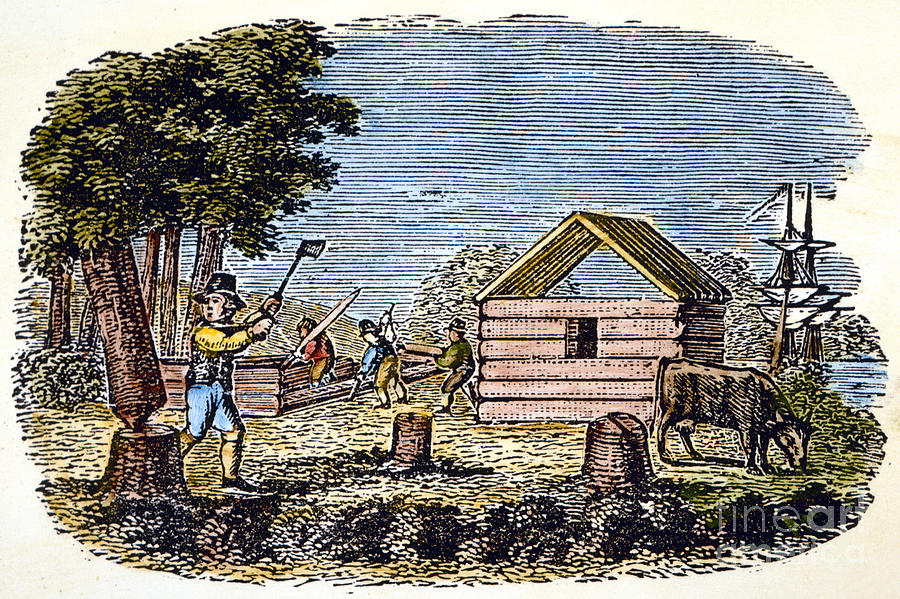This is a detailed illustration, approximately six inches wide by four inches high, featuring a meticulously executed scene that's rich in historical and rustic elements. The background employs horizontal lines in shades of blue, white, and pink, creating a serene, sky-like setting. Surrounding the central image is a faint tea-stained brown border that frames the scene in an old-world aesthetic.

At the foreground, a male figure dressed in a yellow shirt, blue pants, and yellow stockings, and wearing a black pilgrim hat, is diligently chopping down a tree. Behind him, several individuals, similarly attired in early modern period clothing, are engaged in building a log cabin. To the right of this construction scene, another log cabin stands partially completed, featuring a finished foundation and roof rafters.

In the mid-ground, a cow grazes on grass depicted with tiny green dots and lines, adding a touch of rural life to the scene. Past the buildings and parked behind the grazing cow, a bay of water is visible with a tall ship anchored, its sails down, signifying the recent arrival of the pilgrims.

Throughout the image, the artist's technique of using intricate lines and dots helps to build a tapestry of pioneer life, merging both labor and landscape in an evocative portrayal of early settlement.